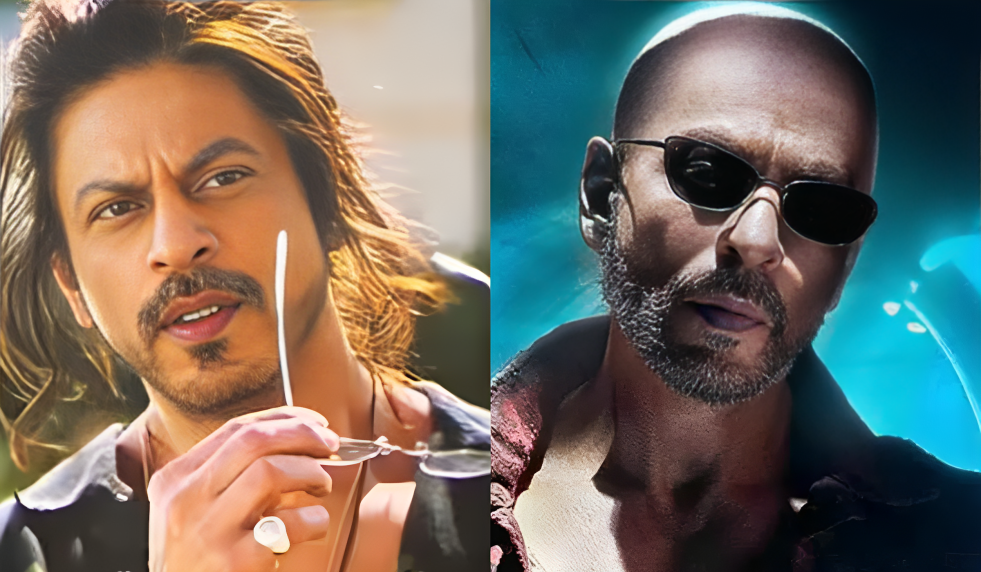The image consists of two AI-generated but realistic-looking portraits of men, side by side. 

On the left, the man has long, flowing dark brown hair, dark skin, and arched eyebrows. He sports a mustache and a goatee, and is squinting slightly while looking away from the camera. He holds a pair of glasses in his hand, revealing a ring on his pinky finger. His attire is a dark-colored shirt, and the background is blurred, suggesting an outdoor scene.

The man on the right is bald with a short, graying beard and mustache that still retains some darker tones. He wears black sunglasses and a red collared shirt that is open at the neck. The background behind him is a blue, futuristic setting that darkens towards the upper right corner, providing a stark contrast to his stern demeanor.